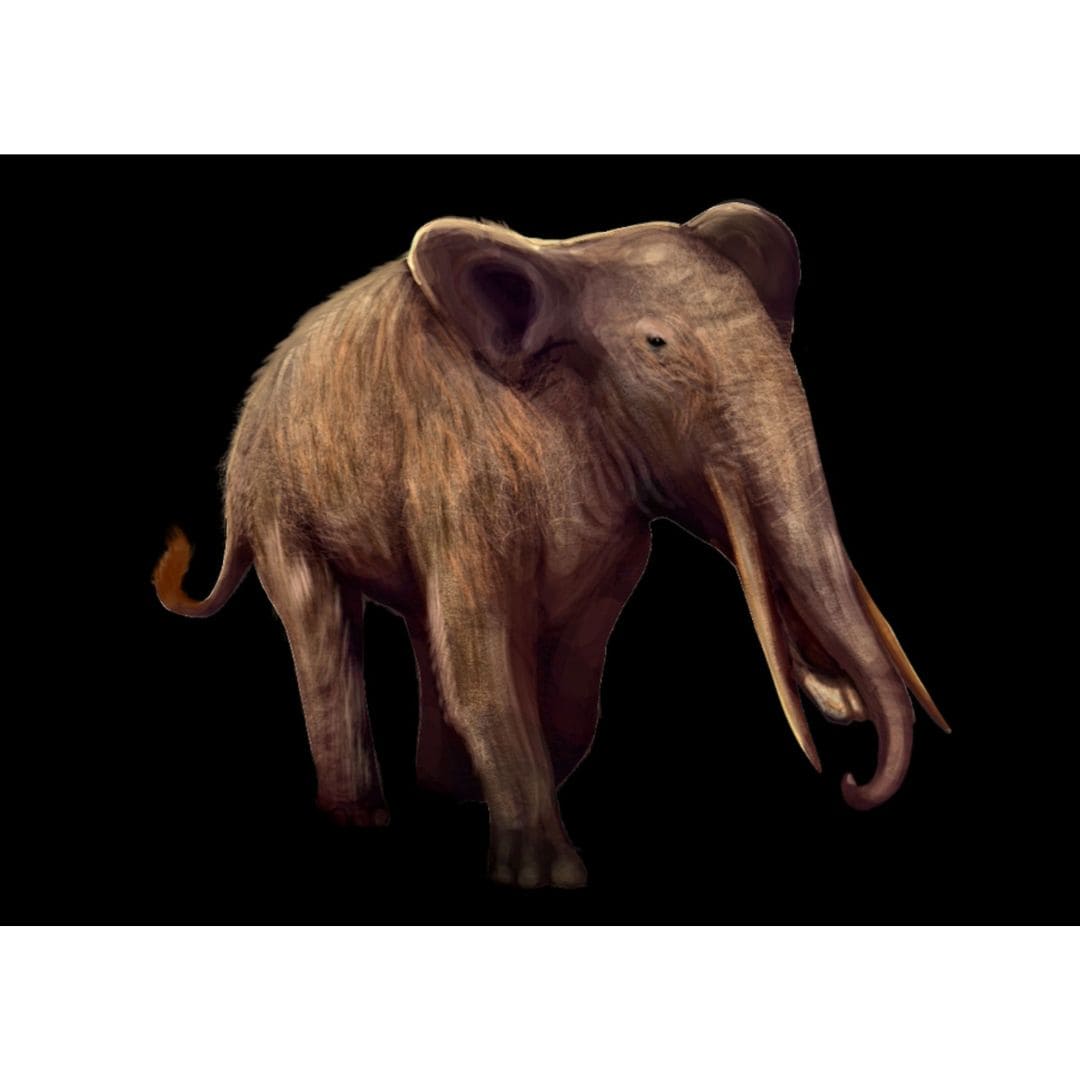This digital rendering depicts a brown prehistoric elephant set against a stark black background. The elephant’s distinct features include a smoother, longer face, and a narrower trunk that tapers to an end. Its tusks, brownish in color, extend downward from the face, reaching almost the length of the trunk. Unlike modern elephants, its mouth extends further down the trunk. The creature has small, high-set black eyes and large ears that are not as floppy as those of contemporary elephants, with the inner ear being darker. Brown fur or hair covers its legs and back, giving it a somewhat fuzzy appearance, with individual strands visible. The elephant appears to be walking, with one leg placed in front of the other, and has a small brown tail. The overall scene captures a detailed view of the elephant in profile, looking towards the right.